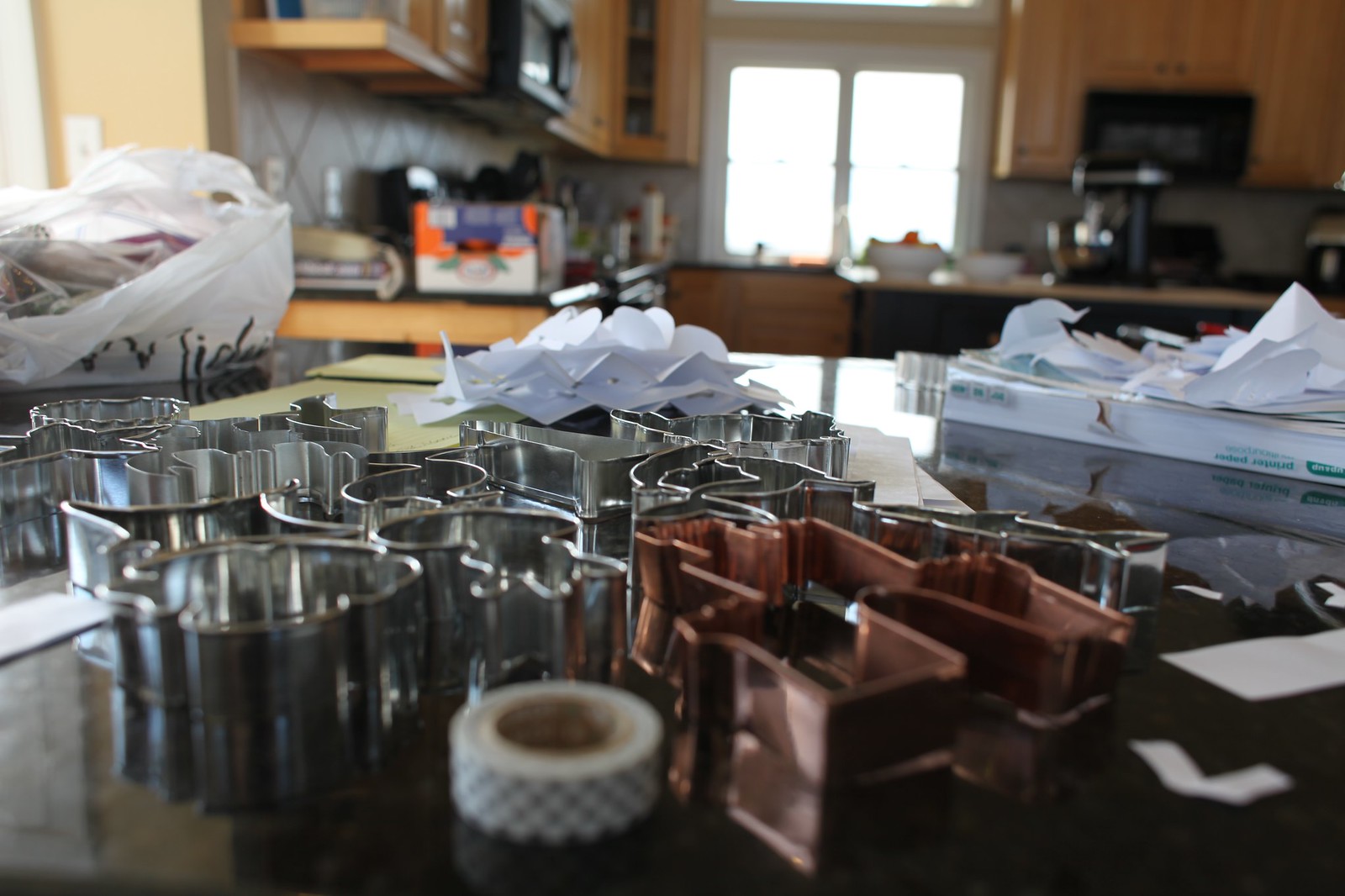In a warmly lit kitchen, the foreground showcases a shiny black surface adorned with an assortment of cookie cutters. Approximately 10-15 cookie cutters, primarily silver with one distinguished copper piece, are scattered across the surface. Among them lies a small roll of white washi tape with a black crisscross pattern. Behind this culinary display, a piece of paper adds an element of mystery, its purpose not entirely clear. The background reveals a slightly out-of-focus plastic bag and a surface leading to light brown wooden cabinets. Nestled into these cabinets are a black mixer and a built-in microwave, hinting at the kitchen’s modern utility. The walls are decorated with white tiles arranged in a crisscross pattern, contributing to the room's charm. Various other items, including a cardboard box, rest on the countertops, giving the scene a lived-in feel. Despite the lack of clarity on the specific shapes of the cookie cutters, their unique forms suggest they could be anything from character outlines to eclectic designs, enhancing the kitchen's creative and homely atmosphere.